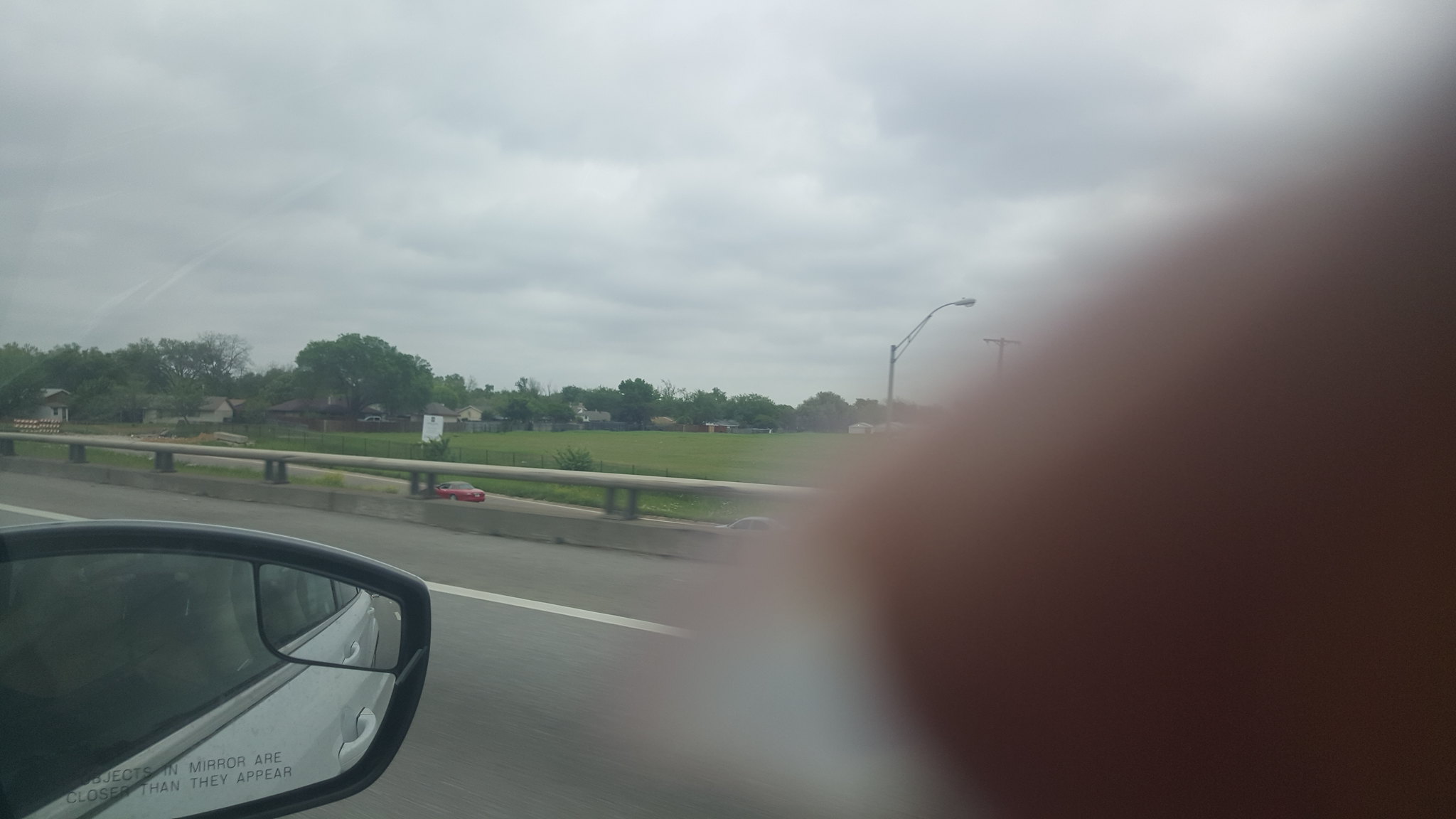This photograph captures a serene moment from a passenger's perspective, taken through a car window. In the bottom left-hand corner, the side mirror with a black outline is visible. Extending from the bottom right to the top right corner is a pinkish-red, sideways triangle, possibly a reflection on the window. The road below the mirror is made of gray asphalt, bordered by a solid white line marking the road's edge. Adjacent to the road, there's a narrow gutter leading to a small gray concrete wall which is topped with a silver circular pole guardrail. Above this scene, the sky stretches across the top of the photograph, exhibiting a tapestry of cloudy gray and blue hues. A line of lush green trees sits below the sky, separated by a stretch of green grass, adding a natural contrast to the built environment.